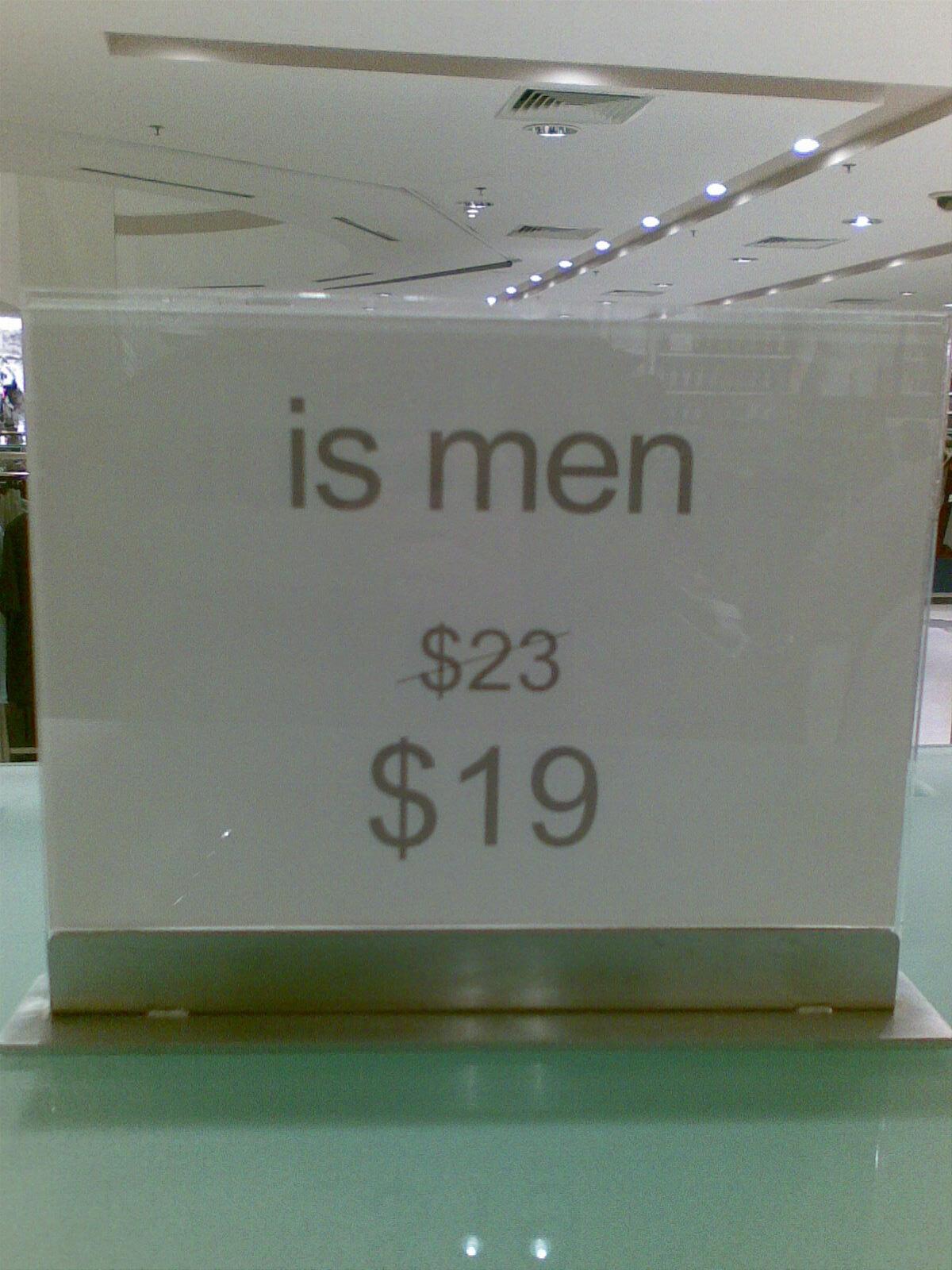In a department store, a display sign is prominently positioned on a smoked glass tabletop. The sign resembles a small, silver menu holder often found in cafes. It features a plastic insert where a plain piece of white paper is slid in. The top of the paper has the text "IS men" written in lowercase letters. Below this, a price of $23 is crossed out with a diagonal line, indicating a markdown. The new price, $19, is displayed in a slightly larger font beneath the original price, highlighting the discount.